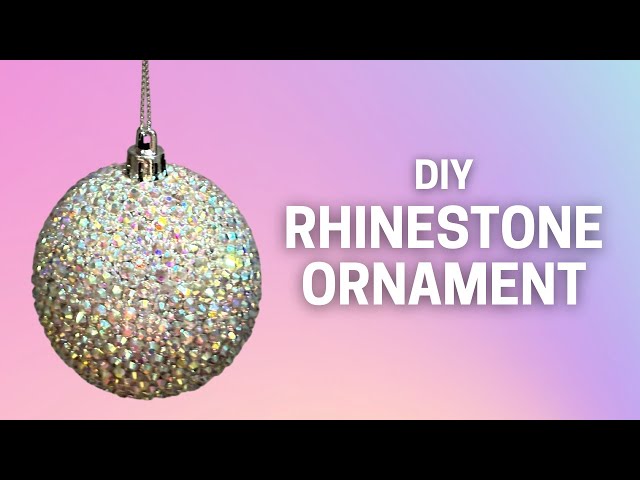The image showcases a dazzling DIY rhinestone ornament with a descriptive text overlay in white that reads "DIY Rhinestone Ornament." The ornament, shaped like a Christmas bauble, is intricately covered in shimmering, multi-colored rhinestones in hues of blue, yellow, pink, orange, and purple, creating a metallic rainbow effect. Its shiny, reflective surface resembles that of a disco ball. The ornament is designed with a bowl shape and a clasp on top, hanging from a metal chain, though the point of attachment is not visible. The background of the image transitions through a gradient of pink, blue, and purple, giving it a dreamy, vibrant appearance, while the top and bottom edges have a black border, framing the colorful display. This appears to be the cover of a project, possibly for a YouTube video tutorial, showcasing the DIY process of creating this sparkling ornament.